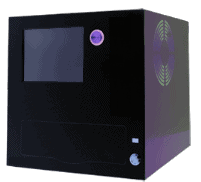The image depicts a large, square-shaped computer tower box, which is a departure from the conventional rectangular design. The tower is predominantly dark in color, with accents of purple and green lighting that seem to emanate from within, suggesting it may contain LED lighting commonly used in gaming or high-performance computers. One side of the box features a visible fan grate, illuminated by both green and purple lights, giving a striking silhouette effect. On the front panel facing the camera, there's a prominent, likely purple power button positioned centrally, which stands out against the dark surface. At the bottom right of this panel, there are a few white stickers, although the text or details on these stickers are indistinguishable. Additionally, the side of the box facing the camera has a panel that appears almost translucent, adding to the unique aesthetic of the tower. Overall, the box is primarily dark gray, adding to its sleek and modern look.